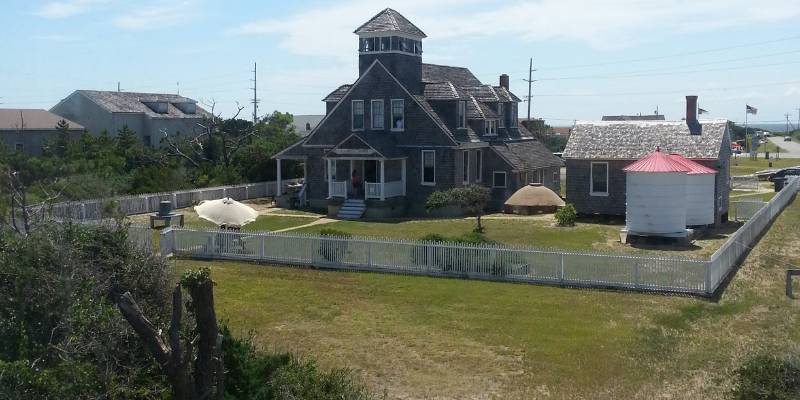This photograph captures an outdoor suburban setting, possibly in Asia. At the center of the image stands an older green house characterized by several windows and a centrally positioned door. Adjacent to this house on the right side is a smaller gray cabin. Encircling the house is a white fence, enclosing a garden area adorned with lush green grass and various plants. Beyond the fence, more grassy ground extends toward the front of the property.

On the left side of the house, and continuing beyond the fence, are several trees and additional houses, suggesting a neighborhood setting. A distinctive feature of the house is a small tower at its top. Blue skies with light clouds loom overhead, adding to the serene atmosphere.

In the backyard, one can observe small sheds with red roofs and an umbrella. There are white stairs leading to the back porch where a woman is present, and a sidewalk that likely connects different parts of the yard. The backdrop of the scene hints at a small town ambiance, complete with mountains, highways, power lines, and well-kept lawns.